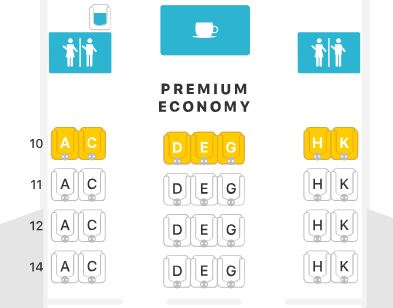The image showcases a premium economy seating layout from Flight Options, focusing on rows 10, 11, 12, and 14. The background of the image is predominantly white, accented with light gray at the borders and some scattered blue and gold hues. Each row is marked by gold-colored labels indicating the seat positions: A, C on the left side and D, E, G, H, K on the right, suggesting a high-tier seating category.

Outside the central white square, numerical labels for the rows (10, 11, 12, and 14) align vertically on the left. Within the square, icons representing a seat and stick figures of a man and woman flank a coffee cup symbol set against a blue background. This icon arrangement implies amenities available in this seating class.

Beneath these icons, the text "PREMIUM ECONOMY" is prominently displayed in bold, capital letters. The seating rows themselves are visually organized, with gold backgrounds for premium seats in rows 10, 11, 12, and 14, contrasting with the white backgrounds of standard economy seats in the rest of the chart.

This detailed representation suggests an elevated travel experience in the premium economy section of Flight Options, distinguishing itself through color coding and strategic icon placement.